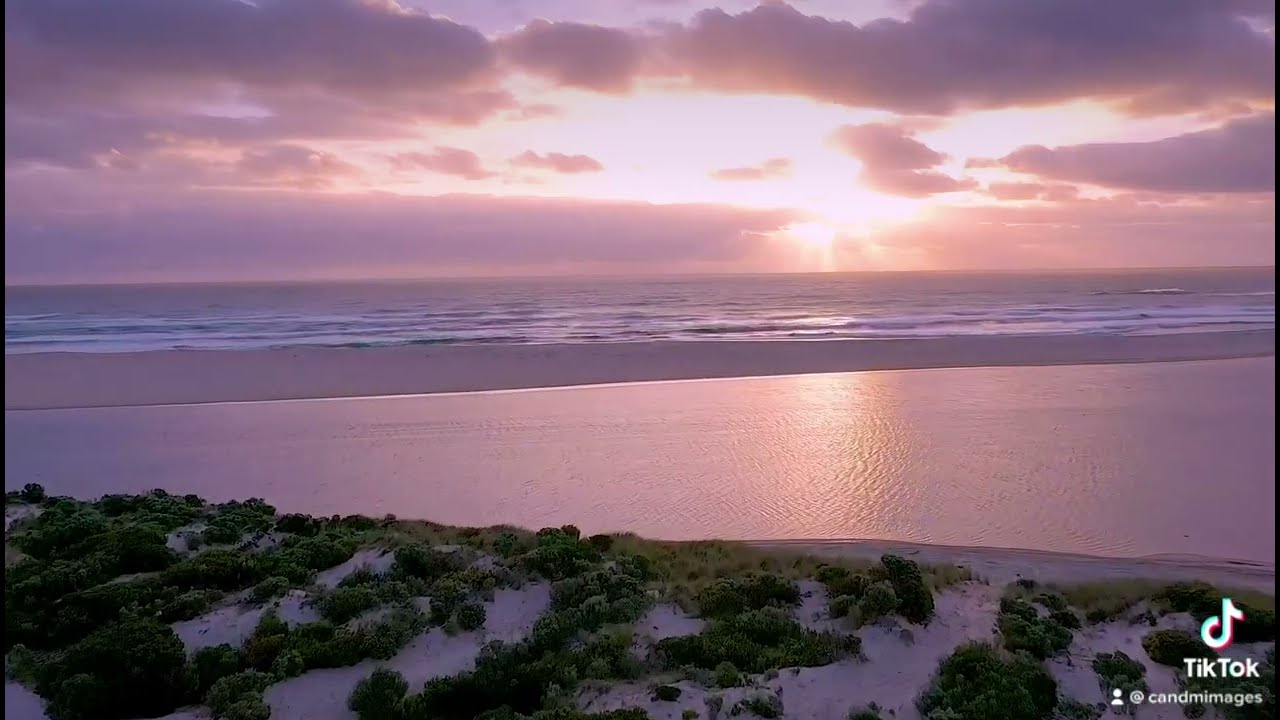The image showcases an expansive and serene beach scene, captured outdoors. The bottom quarter of the photograph features a sandy beach interspersed with smaller bushes and beach grass. Above this sandy expanse, there's a stretch of smooth, flat water, followed by waves crashing near the horizon. Beyond the waves lies the open ocean extending to the horizon line. The sky overhead is filled with a blend of clouds in purples, pinks, and peach hues, reflecting off the water and giving it a distinctive pinkish tint. The sun is setting slightly to the right of the center, casting a warm glow on the scene. In the background, houses dot the largely undeveloped landscape, which is covered with numerous trees and shrubs. The bottom right corner of the image includes a TikTok logo and the handle "@CANDMAGES" written in white. Overall, this tranquil coastal vista, likely reminiscent of a Hawaiian beach, is bathed in sunlight and rich with natural beauty.